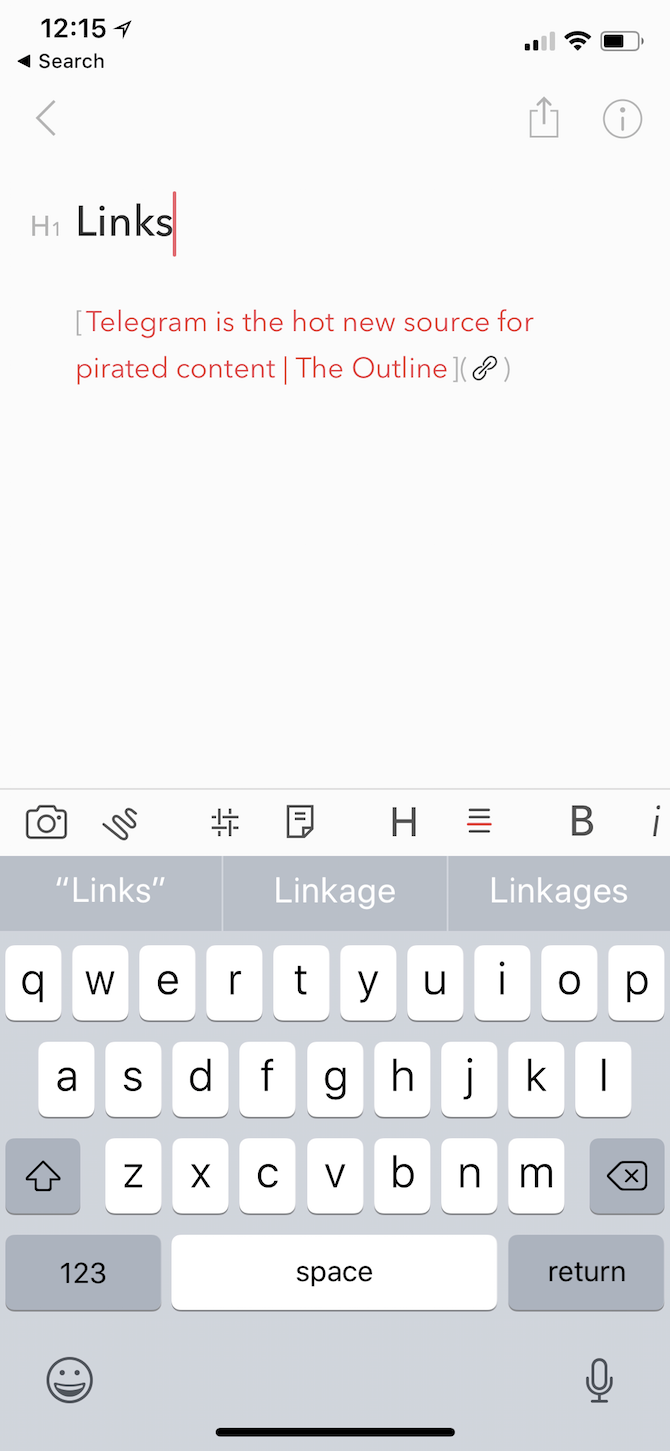The screenshot depicts a messaging application interface where a user is composing a message. In the top left corner of the image, the time is displayed as "12:15" in black text on a white background. The top right corner features several icons: a "204" data connectivity icon, a full Wi-Fi signal icon, and a half-full battery indicator all in black.

Just below the status bar, there is a search bar on the left with a gray left-pointing arrow, an icon resembling a box with an arrow for downloading, and an eye in a circle for additional information or help.

The text area contains the phrase "each one links." The word "Links" is bolded and accompanied by a vertical red line beside it. Following this, text in gray brackets reads: "Telegram is the hot new source for pirated content." This text is highlighted by a red outline and features an infinity chain link logo, indicating a hyperlink.

Further down, there is a toolbar with a camera icon for attaching images and various formatting options for the text, such as bold or italicized style. Below this toolbar, the text "links, linkage, or linkages" is written to illustrate examples of the word.

At the bottom of the screen is a standard QWERTY keyboard layout, complete with emoji icons located at the bottom left and a microphone icon at the bottom right for voice input.